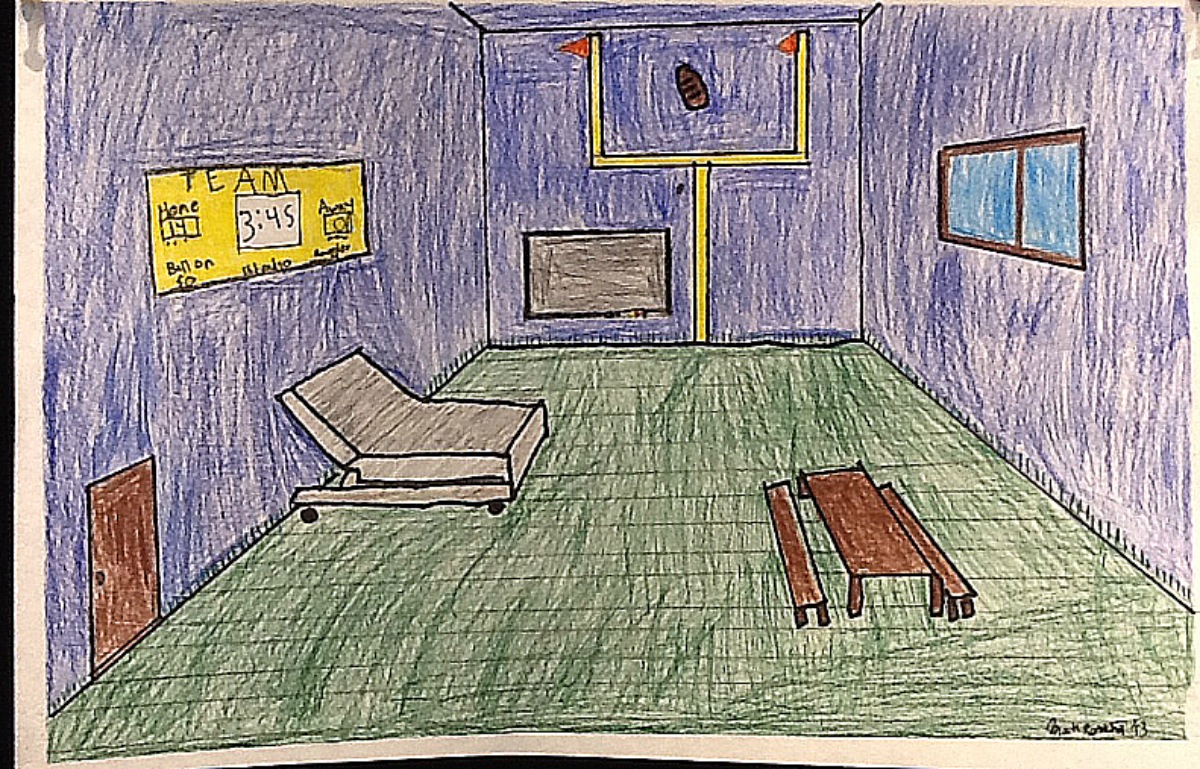A colorful sketch resembling a children's elementary school drawing depicts a well-detailed gymnasium. The gymnasium features a vibrant green floor and striking purple walls. On the right side, a window with a brown frame reveals a blue glass pane, adding to the whimsical color scheme. Within the room, there's a grey bed providing a contrast to the vivid surroundings. A long, brown picnic table-like structure stretches across the space, and a matching brown door can be seen on the left side, enhancing the room's functional design.

On one of the walls, a prominent yellow sign catches the eye. It displays "Team Home 14 Away 0," with a white clock set to 3:45 in the center. Adding to the sporting theme, a yellow football goalpost with small red flags adorns the room, positioned near a brown football placed precisely between the goals. Adjacent to the goalpost is a grey square mounted on the wall, possibly representing a scoreboard or decoration, completing this charming and imaginative gymnasium scene.